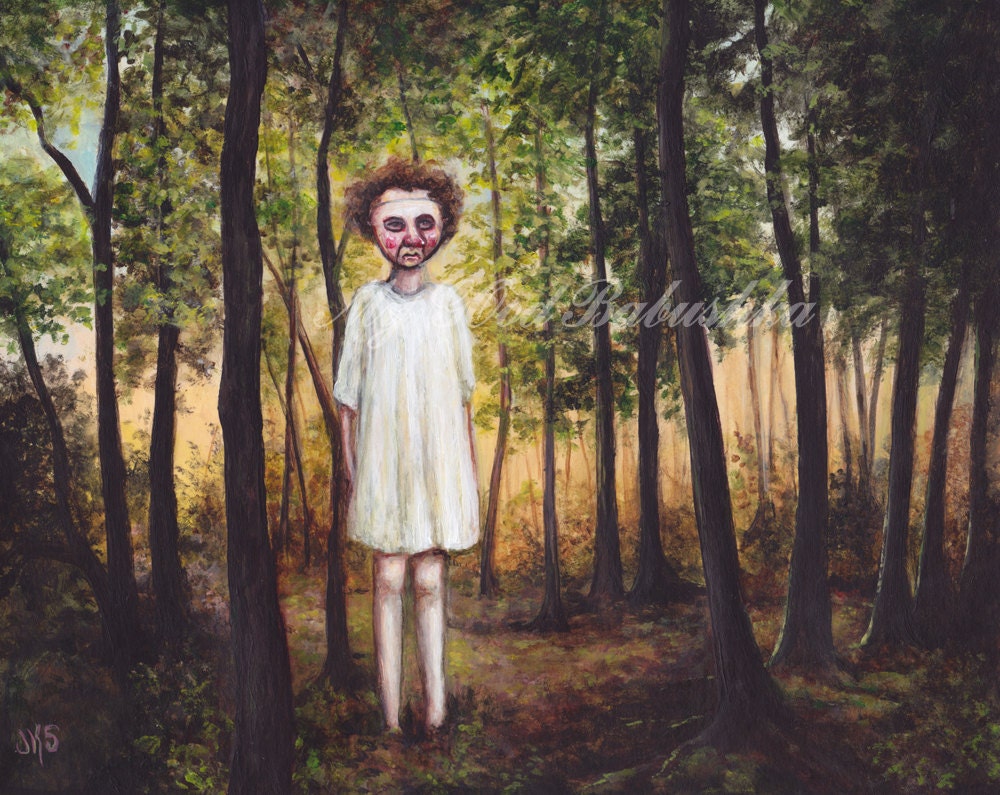This large, square image is a detailed painting depicting a tall, slender human figure standing slightly off-center towards the left in a forest setting. The figure's thin legs, culminating just above the bottom of the image, are very pale and emerge from under a white garment resembling a nightgown that ends just above the knees. They have curly brown hair and a face that is either masked or heavily made up, with prominent pink cheeks and dark brown outlines around the eyes, evoking a somewhat creepy appearance. The faint handwritten text in light gray cursive across the figure's chest reads something akin to "Batusta," though it is difficult to decipher due to poor contrast. In the bottom left corner, the artist's mark "JKS" is subtly visible.

In the background, an array of narrow, dark-brown tree trunks with dark and lighter green leaves creates a dense forest environment. The scene features gaps through which a faint path can be seen winding from the bottom middle to the sides. The sky is partly visible, with a small patch of blue peeking through the upper left corner, while the rest of the background is dominated by a light orange hue that amplifies the eerie atmosphere of the forest.